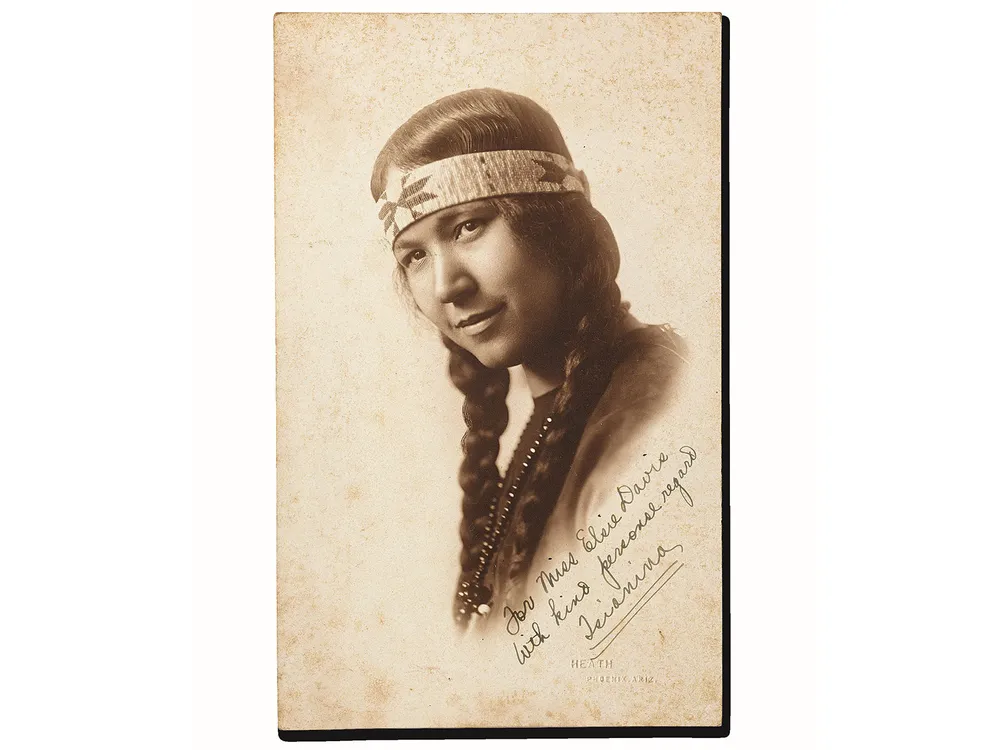This sepia-toned vintage photograph captures a striking portrait of a Native American woman. She is adorned with a headband featuring red markings and wears her dark hair in long braids that fall across her chest. A beaded necklace hangs gracefully from her neck. Her head is slightly tilted to the left, with her chin lifted and gaze directed towards the camera. The backdrop is a worn, tannish hue, with a black border present on the right side and bottom of the photograph. In the lower section of the image, there is elegant cursive text angled horizontally from the bottom left to the right, reading, "For Miss Elsie Davis, with kind personal regard, Sidney Nath." Additionally, the inscription "Heath Photography" is visible in the lower right-hand corner.